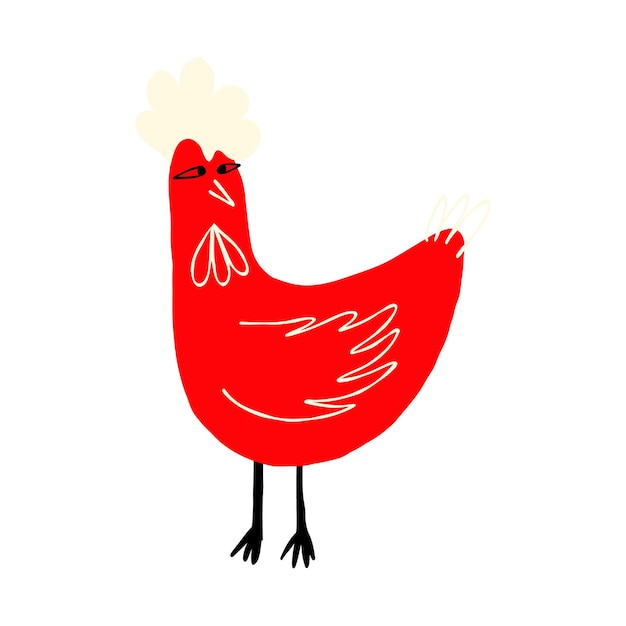This vertical image features a simple, cartoon-like drawing of a red chicken, executed with a magic marker. The chicken's body is arc-shaped, opening upwards, with a taller arc end where the head is located. The chicken's head is very light yellow, almost seemingly with ear-like shapes. It has two horizontal, teardrop-shaped black eyes and a white beak. The chicken possesses three downward-facing white feathers around its throat area. It also has a white wing outlined in white strokes, with three white lines at the tail. The chicken's long black legs are drawn prominently, and it stands facing left, with its head turned back to look towards its wings and outward, creating a dynamic pose. The background of the drawing is completely white, emphasizing the simplicity and bold colors of the chicken.